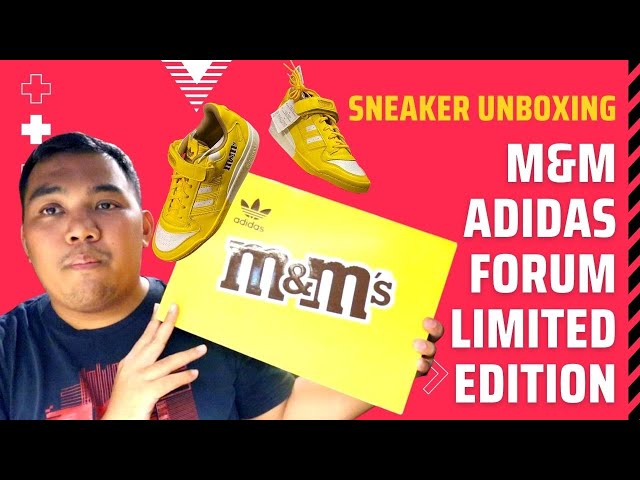This captivating promotional image, seemingly for a YouTube video, features a detailed sneaker unboxing theme centered around a collaboration between M&M's and Adidas. Set against a pink background, the image showcases a young man in a shirt adorned with red graphics, looking directly at the viewer. He is holding a vibrant yellow box prominently displaying the M&M's logo in dark brown, with the Adidas branding situated above it.

To the right of the man, there is a pair of exclusive yellow Adidas sneakers with white stripes and tips, specifically the M&M Adidas Forum Limited Edition. Text on the right side, starting from the top in yellow, reads "Sneaker Unboxing," followed by "M&M Adidas Forum Limited Edition" in white. The entire setup exudes a lively and colorful aesthetic, drawing attention to the unique product unveiling.